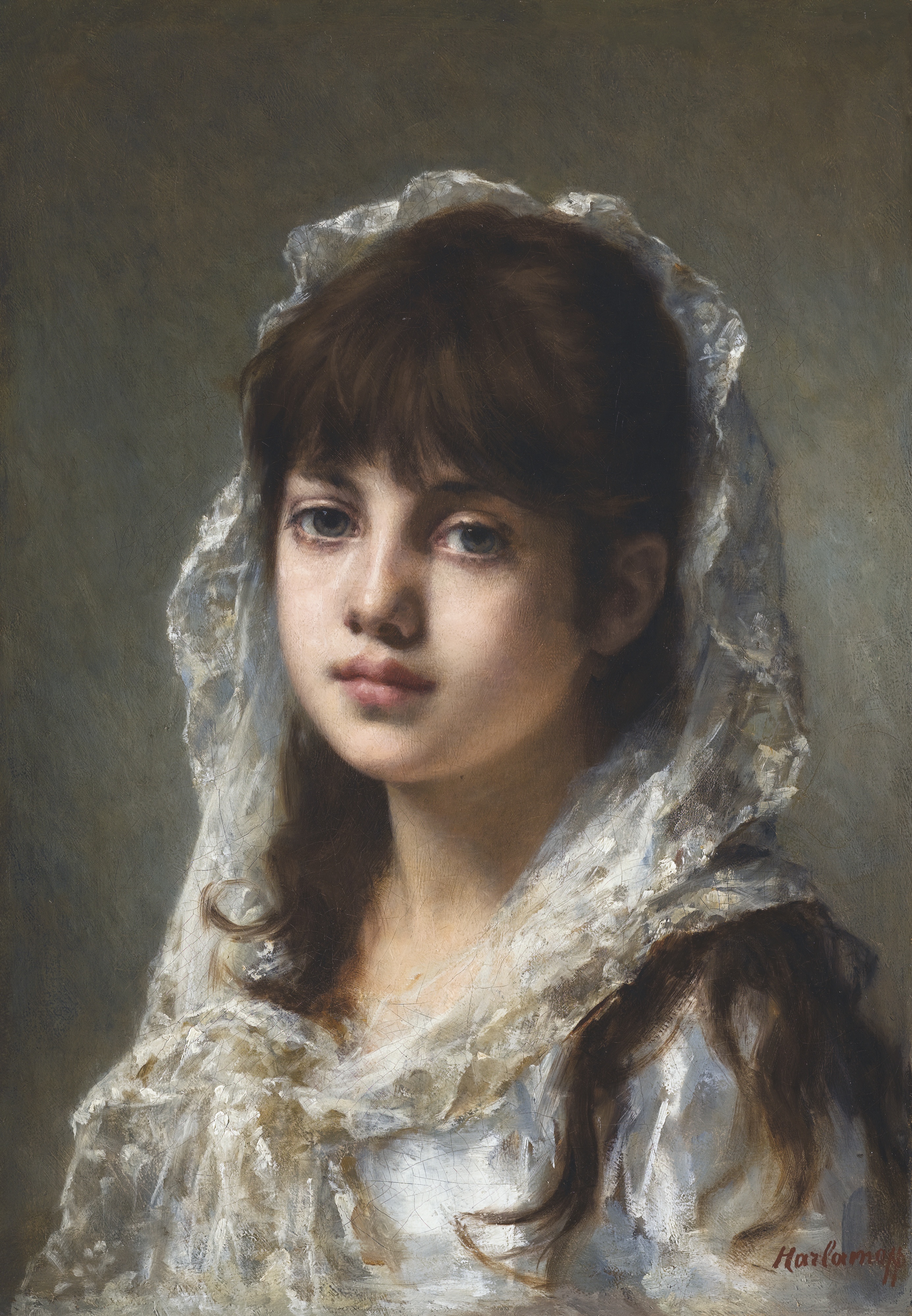The image is an oil painting of a young girl, likely between 12 to 14 years of age, rendered with extraordinary detail and realism. She has long brown hair that extends past her shoulders, with short bangs. She is wearing a somewhat transparent white gown paired with a white veil or head covering, which is tied in a single loop at the front over her chest. The girl's skin is very pale, enhancing the somber expression in her gray or hazel eyes. She is not smiling; her lips are pursed, and she gazes forward with a forlorn look, suggesting sadness or longing. The background is a blend of gray, blue, and darkish green tones, typical of traditional portrait settings. In the bottom right corner of the painting, an inscription in red cursive reads "Harlemoff," presumably the artist's signature. The head and upper torso of the girl occupy most of the canvas, her head slightly turned but mainly facing forward, completing the melancholy yet captivating composition.